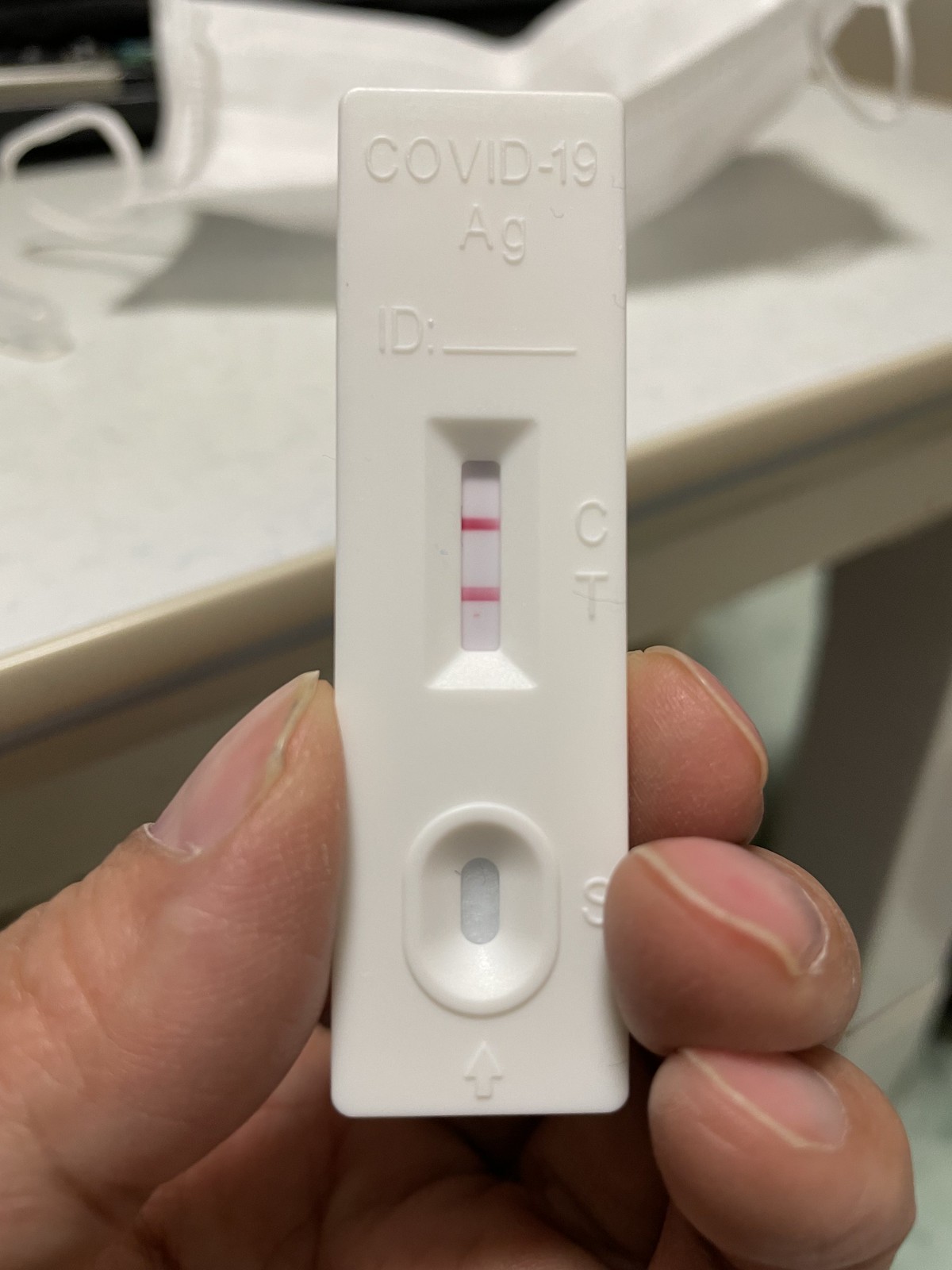This close-up photograph captures a person's left hand, focusing specifically on their four fingers. They are holding a vertical, white rectangular plastic object, which prominently features the text "COVID-19" repeated twice at the top. Below this text is an underscored bar labeled "ID:". The centerpiece of the photograph is a small rectangular viewing window with beveled edges, through which a white background can be seen. Within this window, two small horizontal red bars are visible, positioned apart from each other. To the right of these bars, the raised letters "C" and "T" are displayed in white. At the bottom of the device is an oval-shaped indentation that descends into another smaller oval, again featuring a white background. Near the bottom, a small arrow points upwards, and to the right of this arrow is the letter "S". The image is sharp, showcasing the details and texture of both the device and the person's fingers.